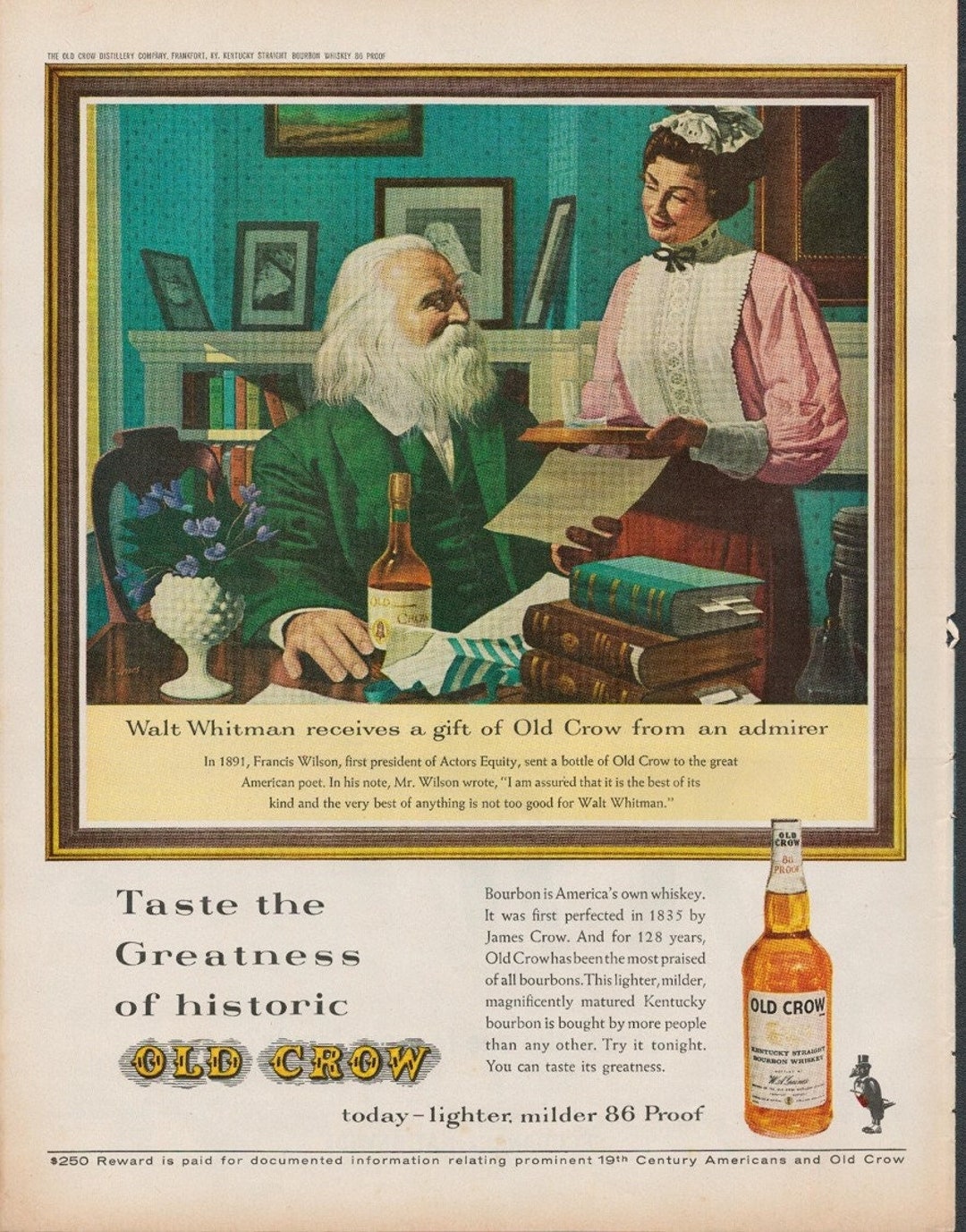This image is an old advertisement for Old Crow whiskey, featured on a yellowed magazine page. Dominating the top portion is a framed, colorful image depicting a scene with Walt Whitman, who appears Santa Claus-like with his long, white hair and beard. Seated at a desk in a green suit, Whitman smiles at a woman standing to his right. The woman is dressed in a pink blouse with a white apron-like lace cover, a red skirt, and a lace-covered hair garment typical of a maid. She holds a tray with an empty whiskey glass, which she appears to be serving to Whitman. 

The setting resembles a cozy study or living room, with stacks of books, a bookcase filled with more books and photos, and a vase of purple flowers in the background. A full bottle of Old Crow whiskey sits prominently on the desk among the clutter. Below the image, text reads, "Walt Whitman receives a gift of Old Crow from an admirer," and smaller text extols the virtues of the whiskey: "Bourbon is America's own whiskey. It was first perfected in 1835 by James Crow, and for 128 years Old Crow has been the most praised of all bourbons," suggesting the ad dates back to around 1963. The bottom right corner features an image of the Old Crow bottle, amber in color, with the text "Taste the greatness of historic Old Crow. Today, lighter, milder, 86 proof."